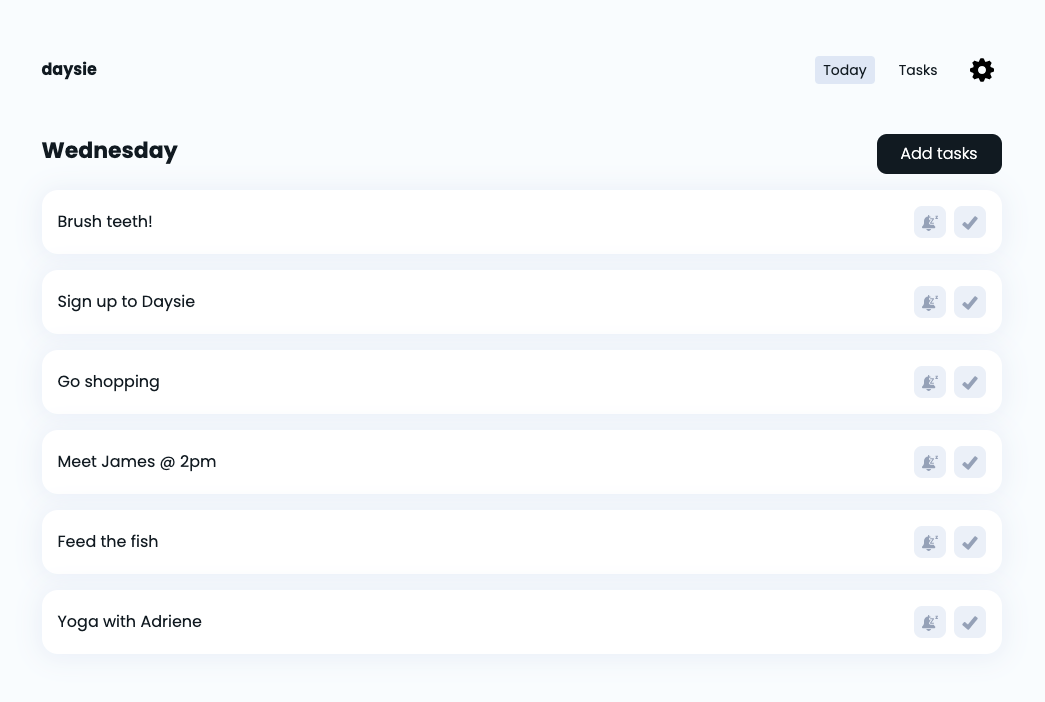In this image, a white background is populated with black text outlining various tasks and settings. In the top right corner, there are several scheduled activities for Wednesday which include: brushing teeth, signing up for Daisy, going shopping, meeting James at 2 PM, feeding the fish, and attending a yoga session with Adrienne. The list appears to function as a daily task schedule for an individual named Daisy.